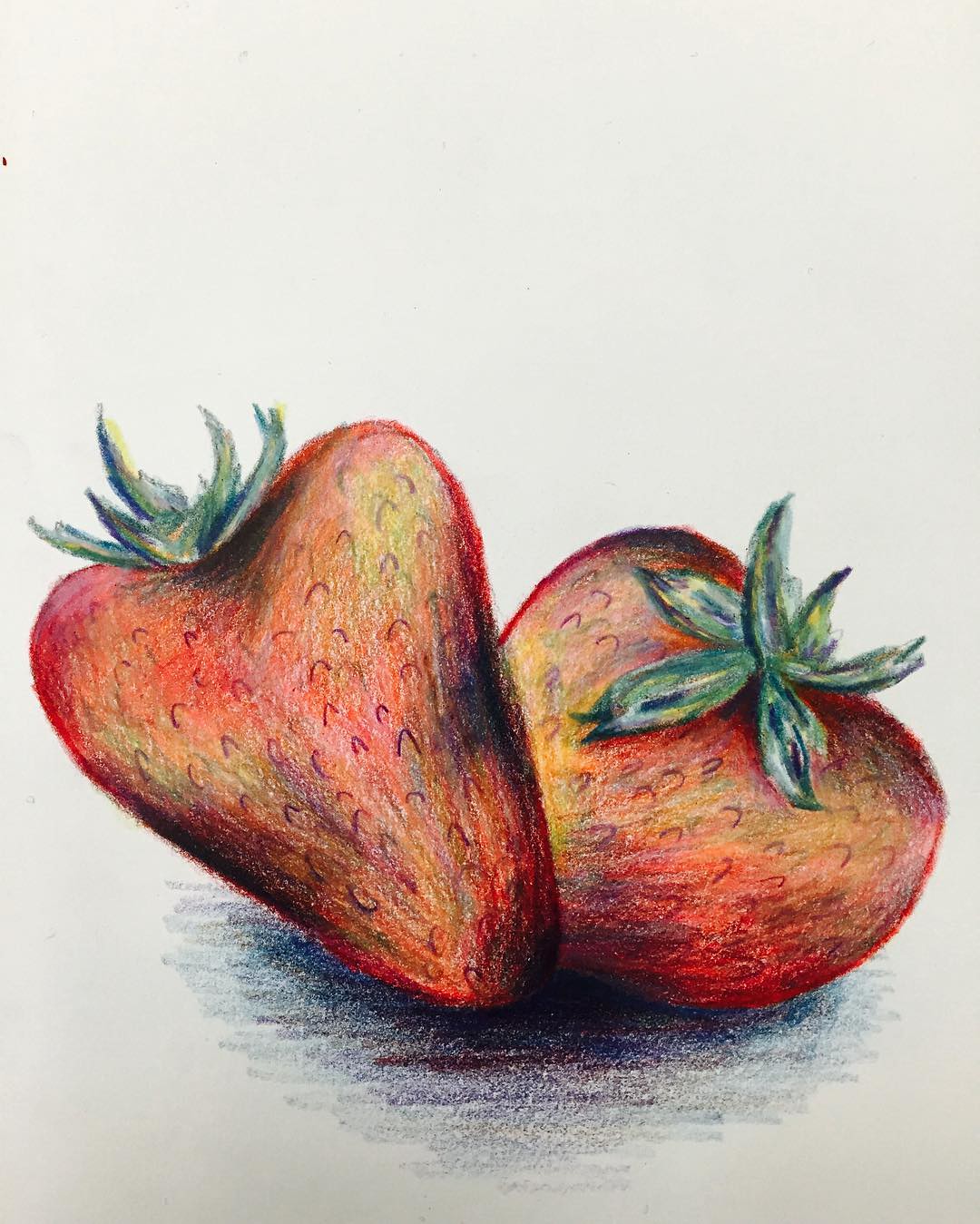This detailed sketch, rendered with colored pencils on a plain white piece of paper with a light grayish hue, depicts two vibrant strawberries against a minimalist background. The strawberries, with their bright red hues mixed with touches of yellow, exhibit a distinct grainy pencil texture. They are positioned slightly overlapping, with the one on the left leaning into the one on the right. Each strawberry is adorned with approximately six to seven small, pointy green leaves on top, pointing upwards and outward from their stems.

The leftmost strawberry, heart-shaped and shaded with a blend of red, yellow, and light green, displays a textured surface marked with small seedy half-circles. The right strawberry, partially obscured behind the one on the left, shows similar detailed texturing and coloration. Both berries feature shadows beneath them, artfully shaded in black pencil to simulate their position on a surface. The overall composition elevates the common fruit into a study of color, texture, and form.